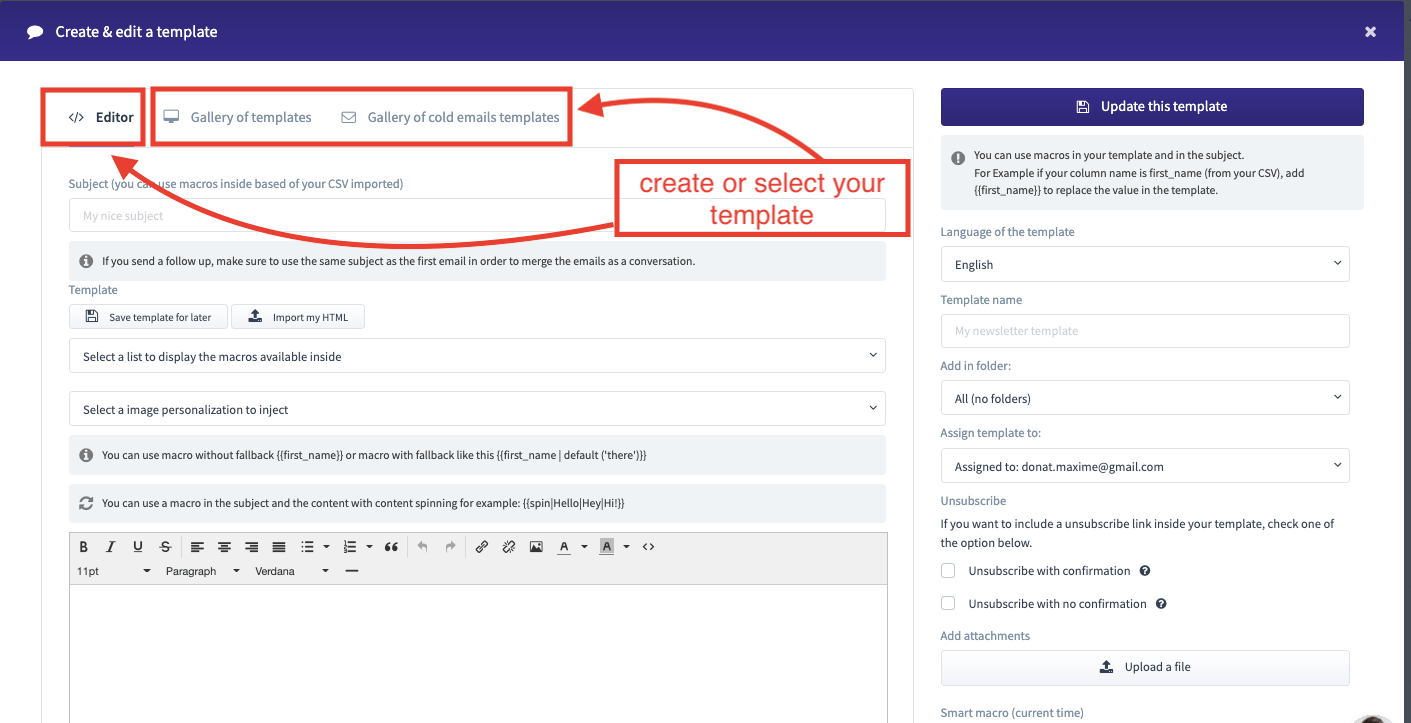The image showcases a user interface for creating and editing a template. The layout is divided into two main areas. On the left side, there is an editor requiring the user to enter a subject name and select a template. Users can add a new template, use an existing one, or import one from another source. Below these options is a section to select a list for displaying available macros, with numerous technical details presented in small, hard-to-read text.

On the right side of the interface, there is a pane dedicated to updating the template, featuring a prominently displayed button. This section informs that macros, which refer to recorded common keystrokes and clicks, can be utilized within the template and subject fields. The template's language is set to English by default, and the template name field must be completed. Additional options include adding the template to a specific folder (defaults to "All") and configuring unsubscribe options, which include checkboxes for "Unsubscribe with confirmation" and "Unsubscribe without confirmation," both of which are unchecked.

The overall background of the interface is predominantly white, with occasional blue accents. Various elements, such as boxes and arrows, are used to direct the user's attention to key actions, such as creating or selecting a template, with one arrow specifically pointing at the "Update this Template" button.